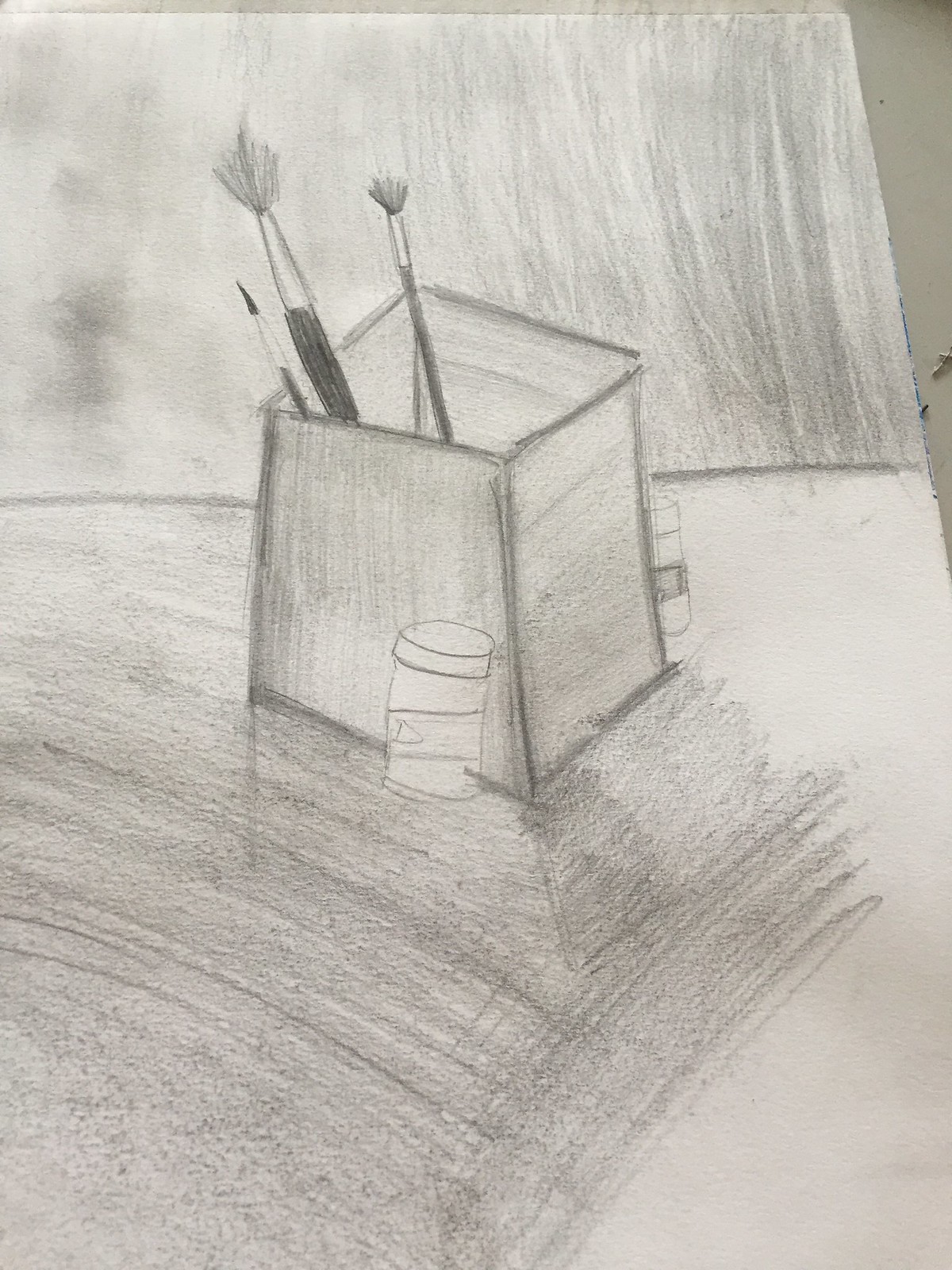This meticulously sketched black-and-white drawing on white paper presents a captivating and detailed still life composition. At the top of the drawing, the artist heavily shaded the area with a pencil, creating a rich gray background. Below this shaded region, a clean horizontal line demarcates the transition to the central focus of the artwork.

Central to the composition is a three-dimensional box depicted with varying perspectives, showcasing the artist’s skill in rendering depth. The box features carefully bordered edges, enhanced by darker pencil outlines for clarity. The box itself appears to be a container holding an assortment of paintbrushes.

The paintbrushes vary in size and detail; on the right, a slender brush with a delicately shaded handle and bristles is clearly visible. To the left, a thicker paintbrush is rendered with equal attention to detail, and beside it, a tiny brush adds to the variety within the ensemble. The brushes are meticulously shaded, with delicate lines indicating the texture and form of the bristles.

Flanking the central box are smaller containers, each outlined and thoughtfully placed to add balance to the composition. The base of the drawing is heavily shaded in gray, simulating the surface upon which the objects rest, though the right side remains less shaded, creating a play between light and dark.

Overall, the artwork is a testament to the artist’s proficiency with pencil shading, attention to detail, and ability to create depth and texture in a minimalist black-and-white palette.